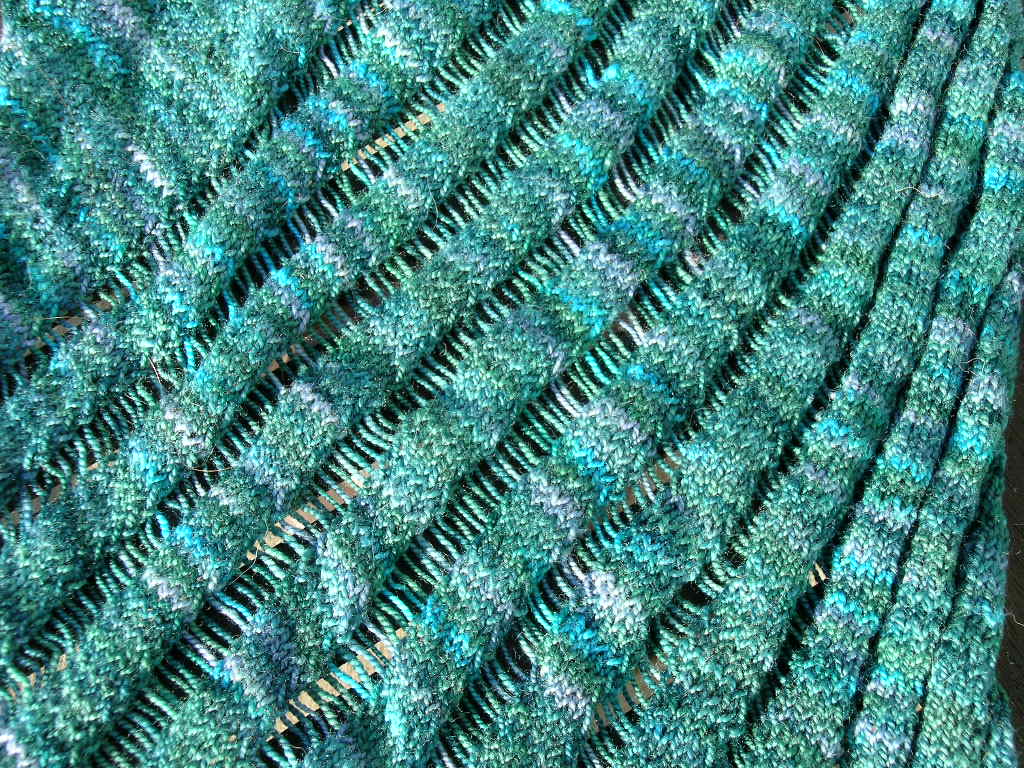This image is an extreme close-up color photograph, captured in landscape orientation, showcasing a highly detailed piece of fabric or woven textile. The fabric is presented in rows set at a diagonal angle from the bottom left to the top right corner. The predominant colors are various shades of blue and green, including light blue, sky blue, teal, aquamarine, and dark green, along with bits of white. The intricate pattern features a herringbone stitch that transitions from light aqua to darker greens and blues. Between each row of stitching, there are open areas with horizontal weaving, adding a fringe effect to the textile. Peeking through these open rows, thin yellow painted lines and some black background details are visible, specifically more prominent in the bottom right corner. Partially visible under the weaving in the bottom left corner are two wooden sticks, likely tools used in the weaving process. The texture and colors suggest an artisan quality, capturing the intricate details and craftsmanship of textile art in a realistic and representational photographic style.